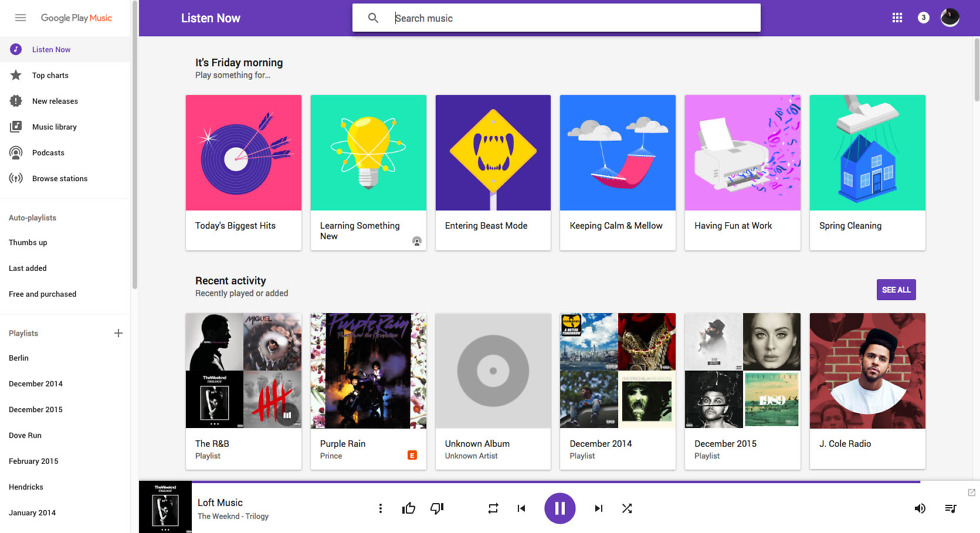**Caption:**

The music webpage features a prominent "Listen Now" button displayed in white with a purple background. This page, dedicated to Google Play Music, includes various sections like "Top Charts," "New Releases," "Music Library," and "Podcasts." The interface highlights the "Listen Now" tab, showing a range of playlists you have created, such as "Berlin December 2014."

Centrally featured, the main section welcomes users with "It's Friday Morning," offering playlists tailored for different moods and activities: today's biggest hits, "Learn Something New" with a light bulb icon, "Entering Beast Mode" with a target and arrows, "Keeping Calm and Mellow" with a hammock hanging in the clouds, "Having Fun at Work" with a printer, and "Spring Cleaning" illustrated by a vacuum attachment.

On the left-hand side, under "Recent Activity," there's a list of recently played items including an R&B playlist, "Purple Rain," an unknown album from December 2014, another from December 2015, and "J. Cole Radio." At the bottom, the currently playing album is displayed with options to like or dislike the song, go back a track, pause, play, or shuffle the music.